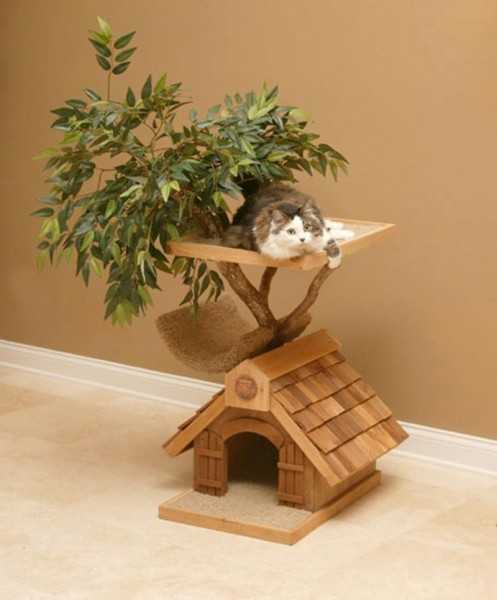This photograph showcases an elaborate and unique cat tree setup in a room with light brown walls, white baseboards, and a beige floor. The cat tree features a wooden base with a light gray carpeted floor, forming the foundation. It resembles a miniature house, complete with small doors and a roof adorned with angled wooden shingles. Attached to the side of this roof on the left is a U-shaped fuzzy platform. From this, a brown tree branch extends at a 45-degree angle, adorned with artificial green, pointy leaves, occupying the top left quadrant of the image.

Adjacent to this setup, a wooden platform extends to the right, where a long-haired cat is comfortably lounging. The cat has a striking appearance, with a large brown body and a white front. Its face is half white on the left side and brown on the right, featuring small green eyes. The cat’s left front paw, covered in white "mittens," dangles off the edge of the platform. This imaginative cat tree design integrates natural elements and cozy platforms, creating a visually appealing and functional space for the cat.